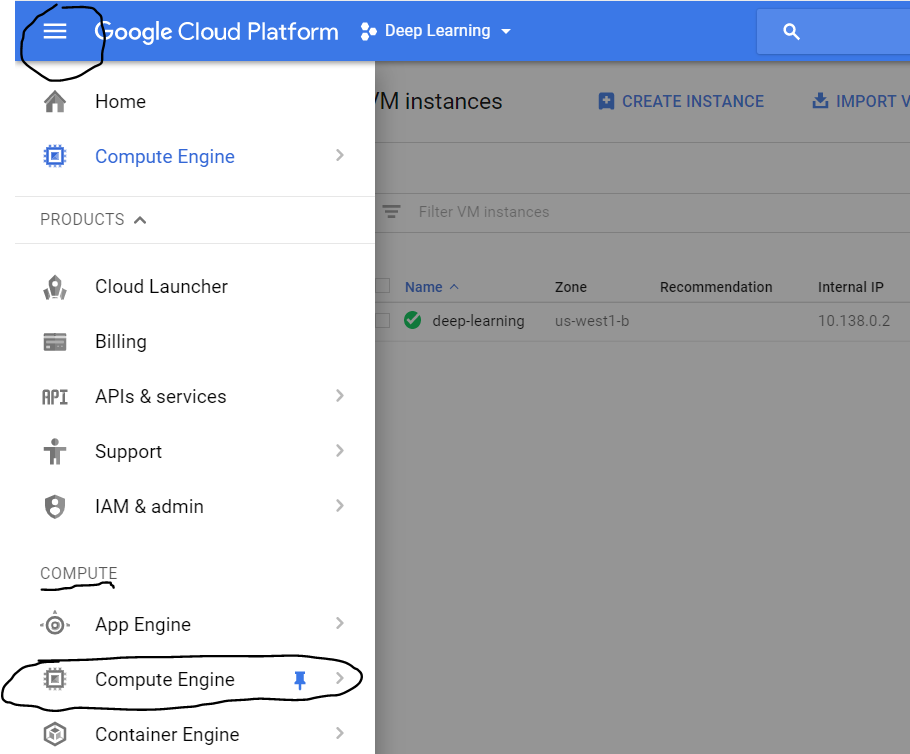This image showcases the Google Cloud Platform interface with a focus on deep learning functionalities. The "New" button is prominently highlighted in black. The left navigation pane displays various menu options including "Home," "Compute Engine," and "Products." Under the "Products" section, you can see options such as "Cloud Launcher," "Billing," "APIs and Services," "Support," and "IAM and Admin." Key sections like "IAM and Admin" and "Compute Engine" are highlighted and seem to be pinned for quick access. In the background, options for "App Engine," "Container Engine," and "VM Instances" are visible. Additionally, there is an open menu for "Create Instance" specifically under "Deep Learning," with the Internal IP address listed as 10.138.0.2. This detailed layout emphasizes the functionalities and tools available for managing and deploying deep learning applications on the Google Cloud Platform.